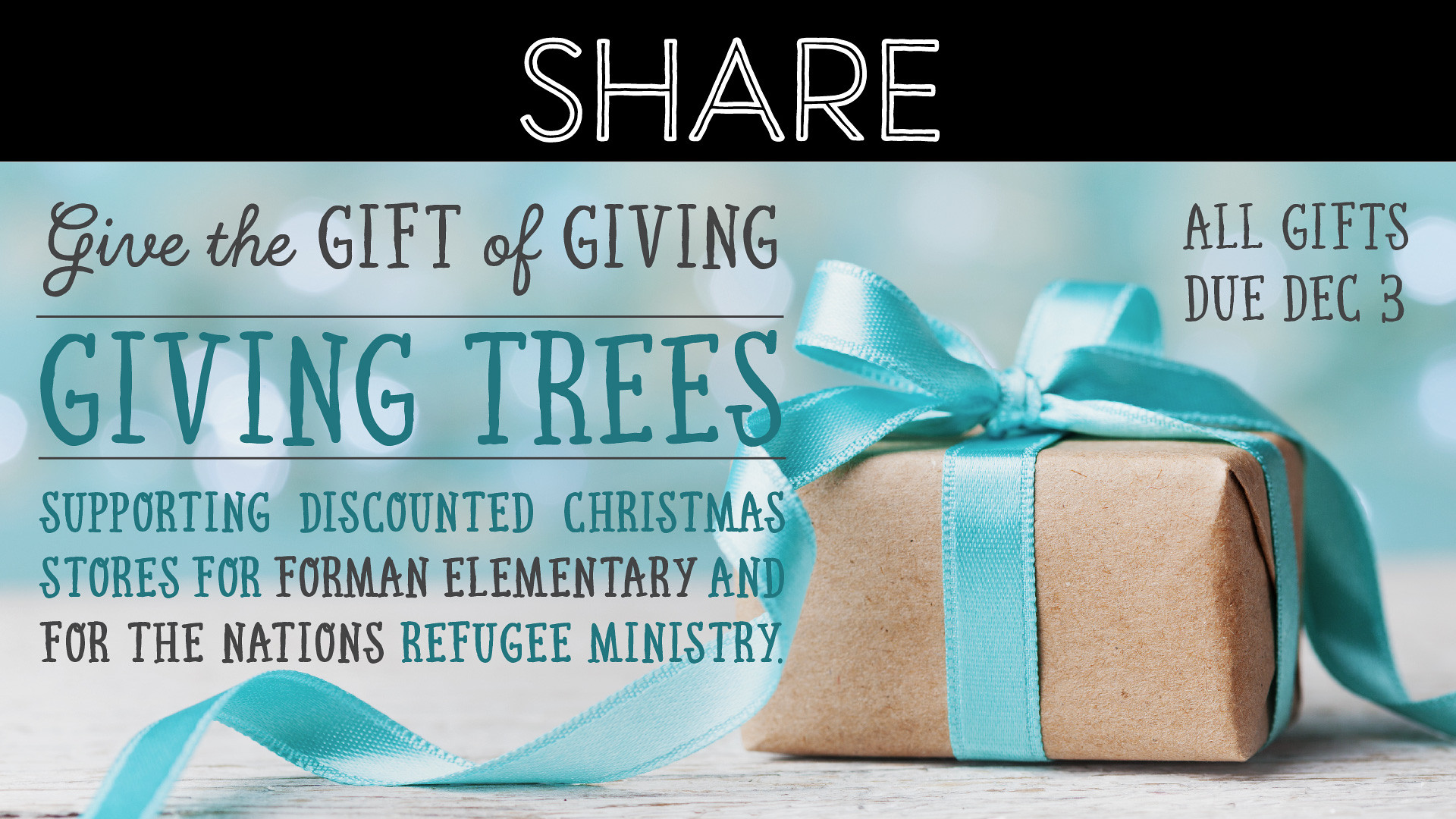The image is a graphically generated advertisement featuring a three-dimensional, rectangular present wrapped in brown paper with a blue bow, resting on a gray, flat surface. The primary background of the advertisement is a pale pastel blue. At the top edge of the image is a black rectangle with centered white text reading "SHARE". To the left of the present, large cursive and bold text reads, "Give the Gift of Giving," followed by, "Giving Trees," in a slightly darker teal color. Below this, additional text states, "Supporting Discounted Christmas Stores for Forman Elementary and for the Nation's Refugee Ministry." Above the present, in smaller black text, it mentions, "All Gifts Due December 3rd." The entire advertisement combines both cursive and bold fonts, and it maintains a delicate pastel aesthetic without traditional holiday colors.